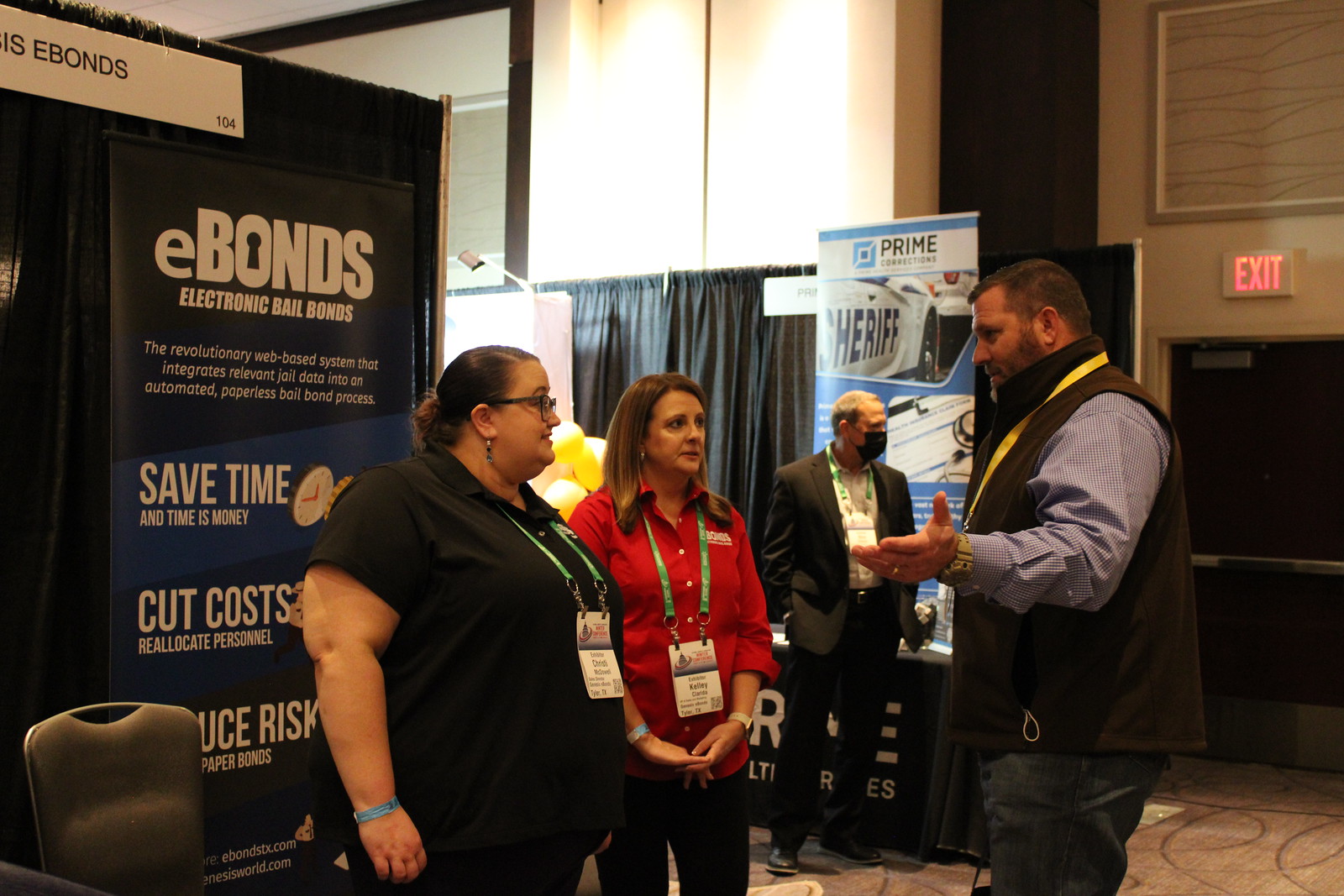This photograph, taken in a dimly lit indoor convention center, shows a group of four people engaged in conversation. They are in front of a door with a red "EXIT" sign above it, to the right of the green-colored wall. On the left side, two women are visible: one in a black t-shirt and the other in a red shirt. Both women have green lanyards with white labels around their necks. To their right is a man wearing a brown jacket and a yellow lanyard, who is talking to them. Behind these three, another man stands, wearing a mask and a plaid blue shirt with a black vest and blue jeans, but he is not actively participating in the conversation.

Surrounding the group, there are several black curtains and multiple posters. Directly behind the woman in the black shirt, a poster reads, "E-Bonds, Electronic Bail Bonds." The text continues vertically with messages like "save time and money," "cut costs," "reallocate personnel," and "reduce risk." In the background, another sign reads "Prime, Sheriff" in blue and white. The environment suggests that attendees are at a convention or business fair, gathered around various informational displays and kiosks.